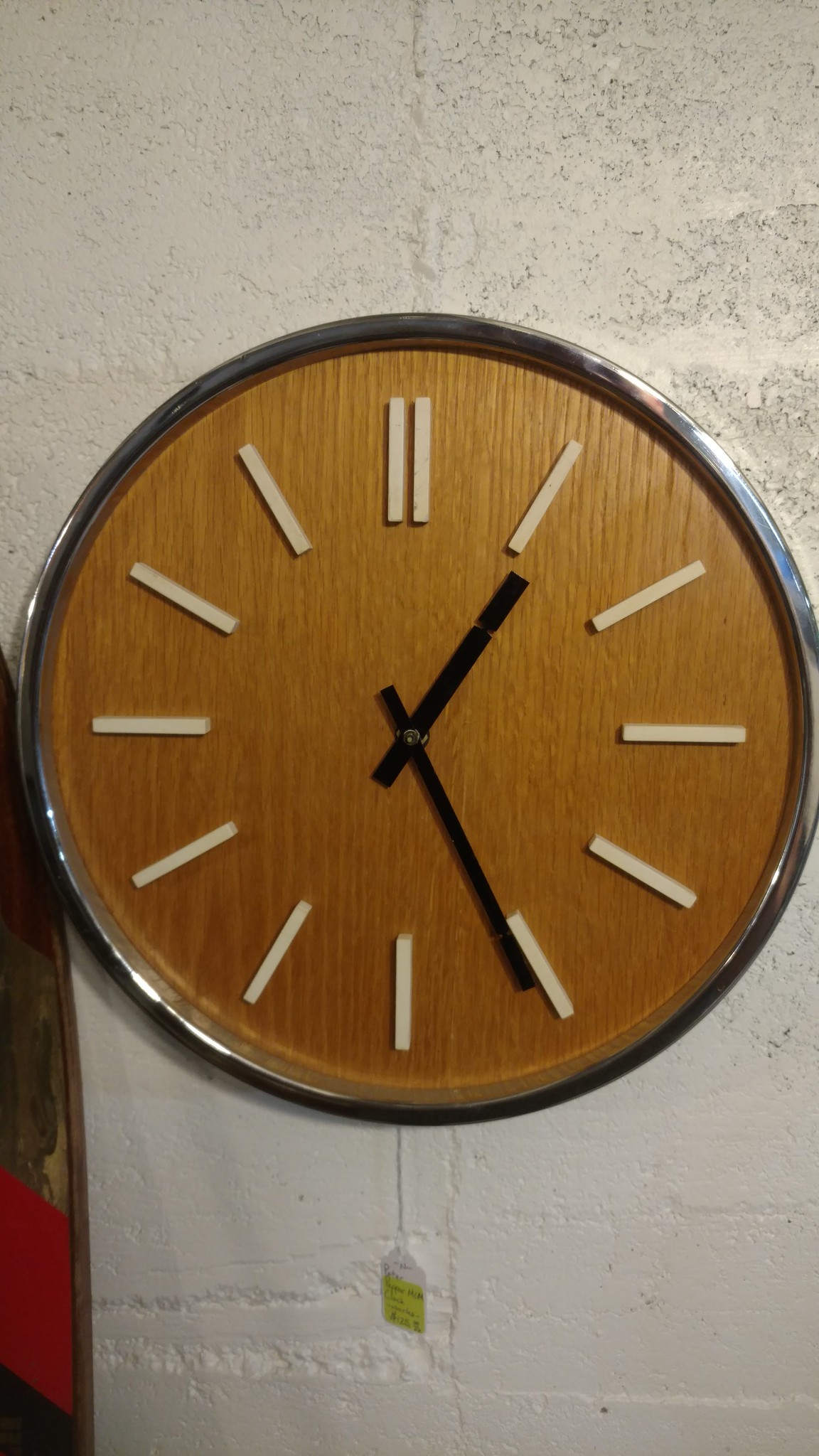The image depicts a modern-looking circular wall clock with a wooden face, featuring a lighter shade of wood. The clock has a sleek silver metal rim. Instead of traditional numbers, the hours are marked by elongated, lighter beige wooden dashes—one for each hour, while the 12 o'clock position is marked by two lines. The clock hands are black, indicating the time is 1:26. Hanging from the clock is a string with a white and yellow sale tag attached, suggesting the clock might be for sale. The background is a white or cream-colored painted concrete wall. On the left side of the image, there is an indistinct wooden object with a red stripe running through it. The clock is prominently centered in the photograph, slightly spilling over the right edge.